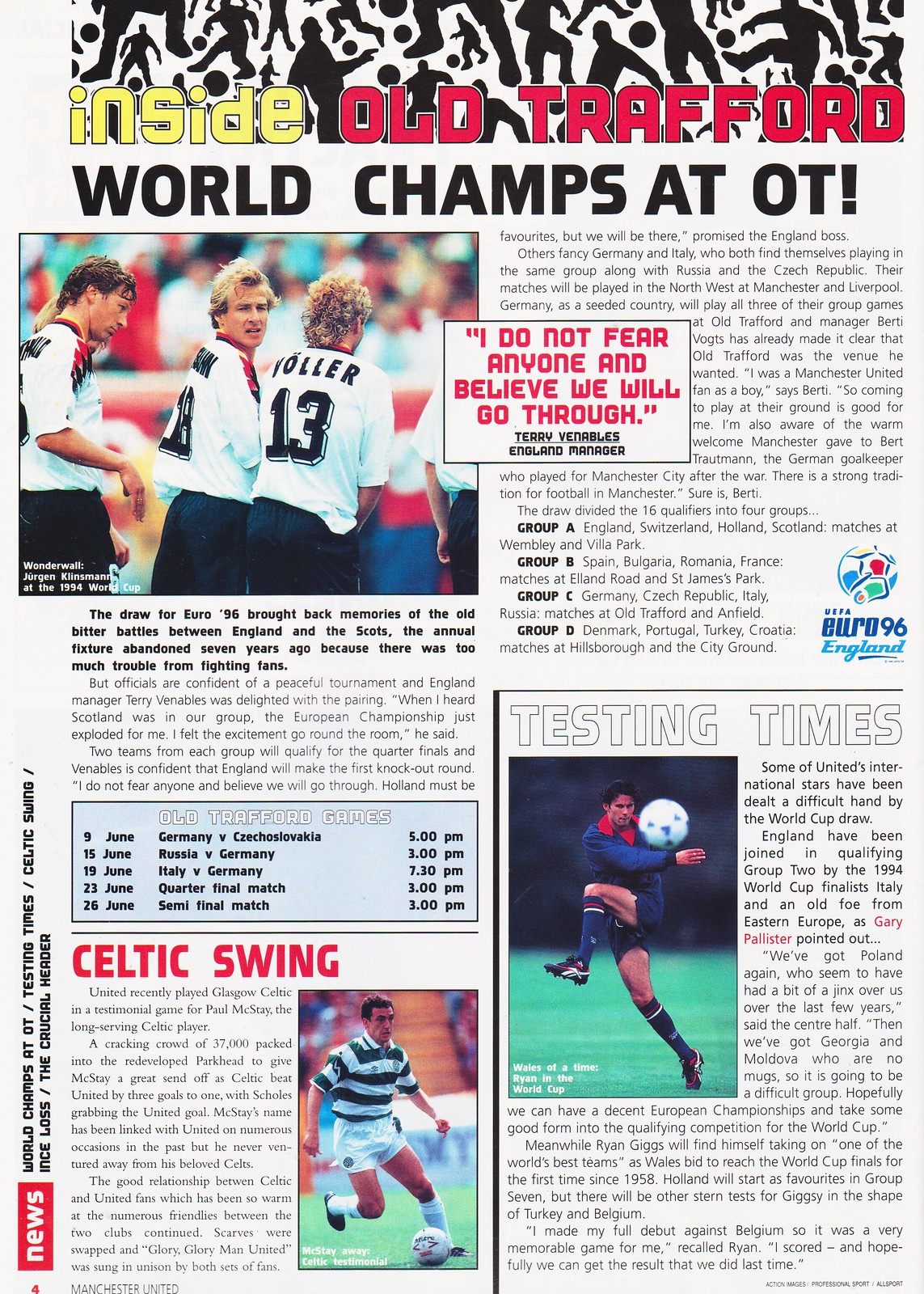The image is a scan of an interior page from a soccer magazine titled "Inside Old Trafford: World Champs at OT," denoted prominently in yellow and red stylized text against a white background. The topmost banner features silhouettes of soccer players in black. In the upper left is a photograph of three players in white jerseys with black numbers: number 13 in the foreground and number 18 behind him, all wearing dark blue shorts. Adjacent to this, in a red box, a quote reads, "I do not fear anyone and believe we will go through," attributed to Terry Venables, England manager.

The left column primarily includes text with an article featuring "Celtic Swing" at its bottom. This section is highlighted in red text and includes an image of a man in white shorts and a green and white striped shirt, standing on one foot with both hands outstretched, kicking a soccer ball.

In the right column at the bottom, there is a section titled "Testing Times," in bold white text with a black outline. Below this is a picture of a man in a blue jersey and black shorts, socks, and shoes, one knee raised high with a soccer ball near his outstretched hand. Additional references on the left mention "Mixed Day Away Celtic Testimonial" and on the right "Whales of a Time: Ryan in the World Cup."